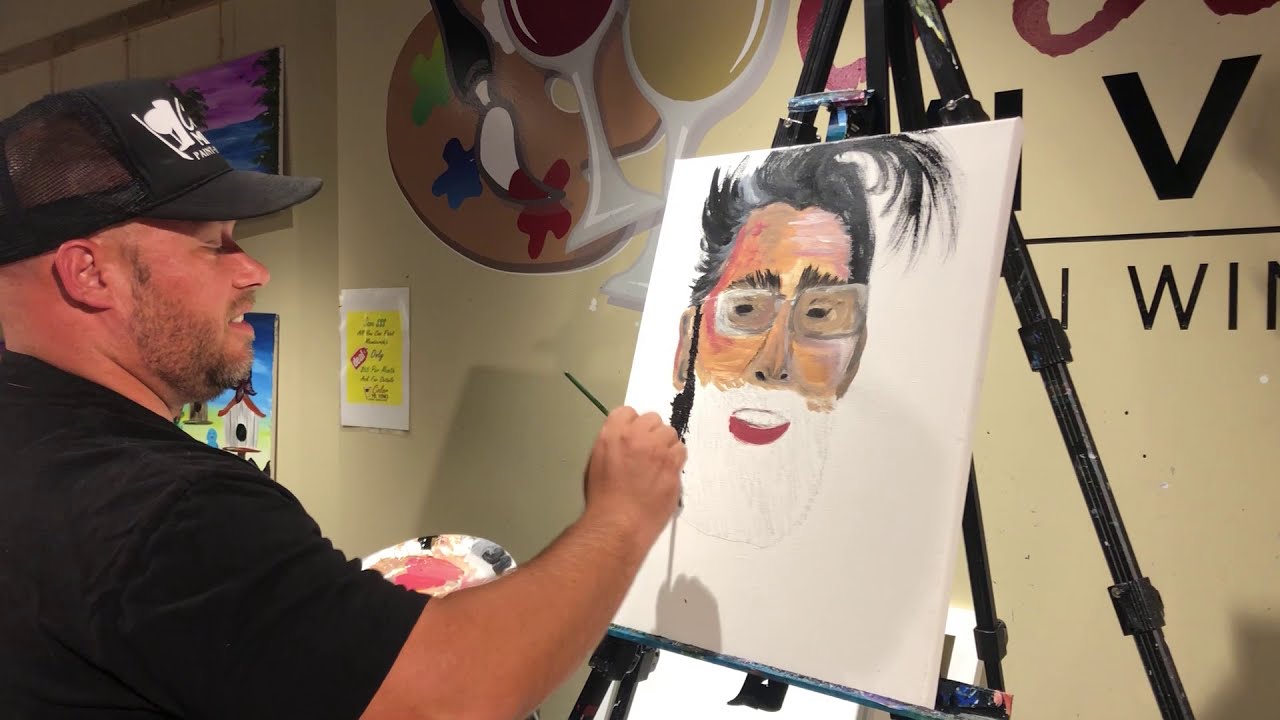In this indoor photograph, the setting appears to be an art studio designed for a wine and paint experience. Dominating the left side of the image, a slightly sunburned, Caucasian man is seen wearing a black short-sleeved shirt and a black trucker-style hat. A thin beard and mustache frame his face. His right arm is extended forward, holding a paintbrush, as he works on a portrait on a white canvas set upon a black easel. The portrait, half-complete, displays the face of a person with swirling black hair, gray glasses, and orangish-yellow skin tones. You can see the faint beginnings of red lips being added to the artwork. To the left of the man, a paint palette is visible, suggesting he is actively mixing colors for his creation. The background features a light brown wall adorned with painter’s palettes and a couple of wine glasses, reinforcing the idea that this is a relaxed, social environment for creating art. Vibrant hues of black, white, purple, yellow, green, gray, blue, and brown contribute to the lively atmosphere captured in the photograph.